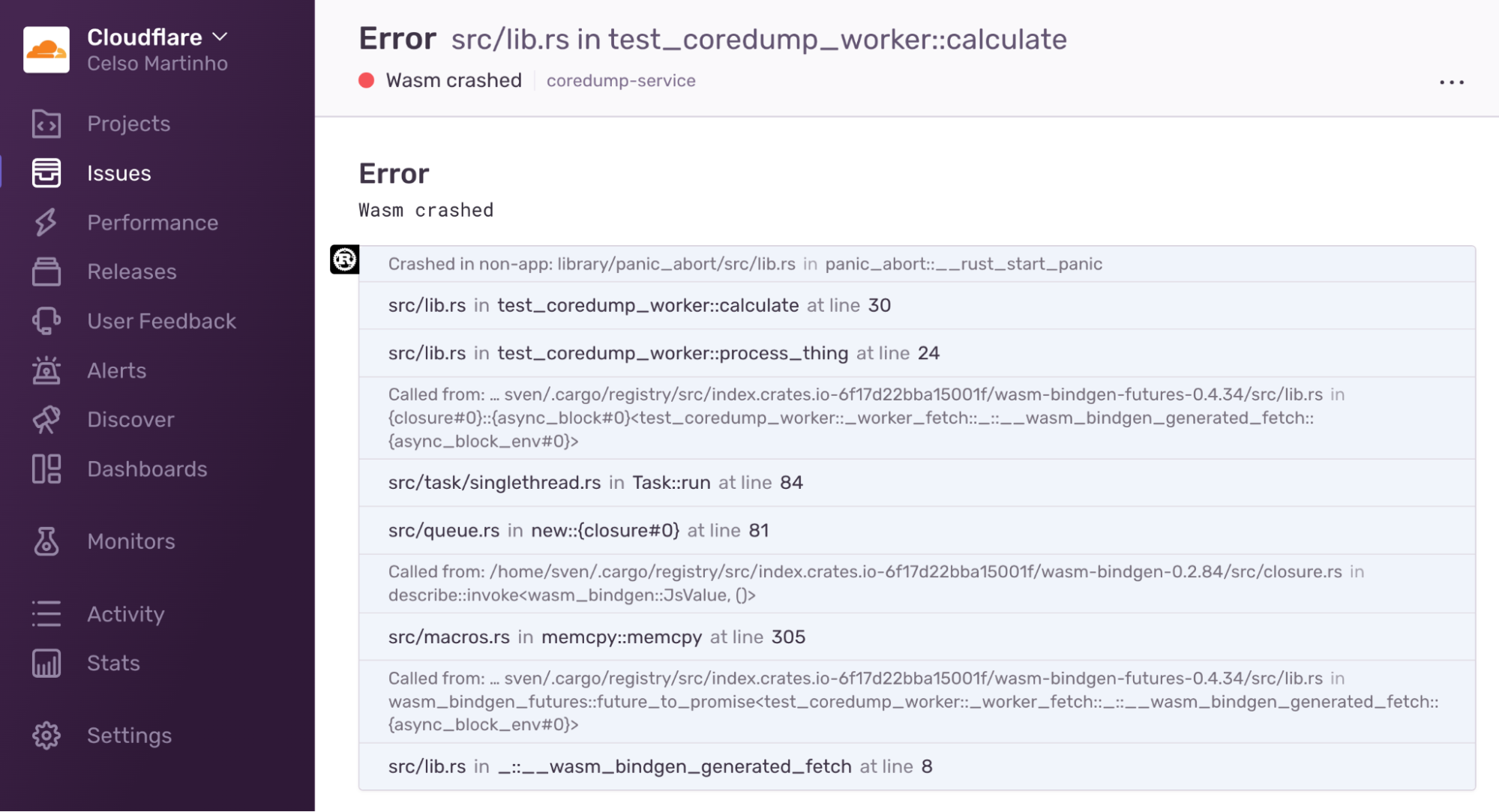The image is a color screenshot in landscape orientation of a CloudFlare application interface. The left side features a vertical, black navigational panel with a white square containing an orange cloud icon, next to which are the words "CloudFlare" in white text. Below that, the account name "Celso Martinho" is displayed, followed by a list of navigational buttons in light gray— the second of which, labeled "Issues," is highlighted in white.

On the right side of the screen, an error message at the top is presented in bold black text. Directly underneath, an orange dot followed by black text reads "WASM crashed." A URL is visible at the top of this section, followed by the word "Error" and a light gray area displaying URL information and reference numbers. The error message details that the issue is in the script located at "src/lib.rs in test_core_dump_worker::calculate," indicating a problem in Celso Martinho’s app scripting that led to a WASM (WebAssembly) crash.